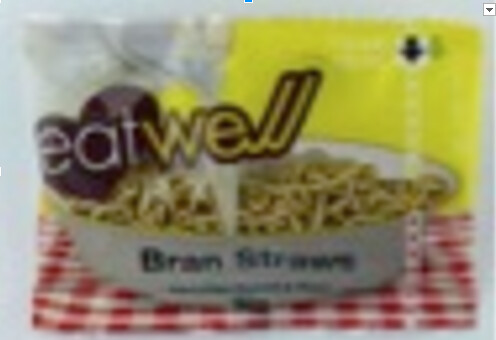In the image, there is a packet of food, likely noodles or bran flakes, displayed prominently against an old-style red and white checkered kitchen cloth. Despite the blurriness, the packet's top is a blend of white and yellow, with the brand name "Eat Well" clearly visible, promoting a message of healthy eating. The dish containing the food is white, and although the labeling is indistinct, the word "bran" can be deciphered, suggesting the product might incorporate bran elements.